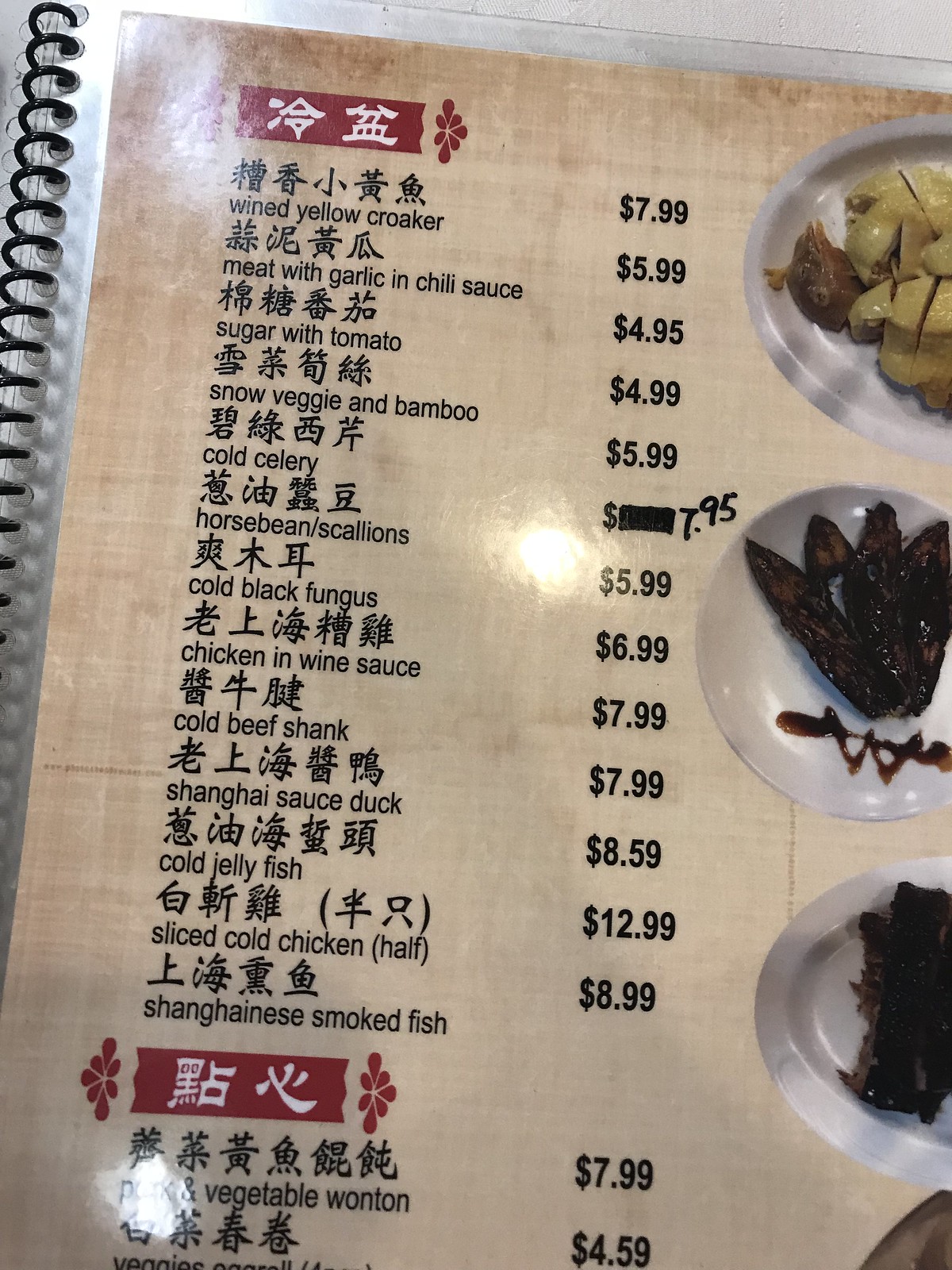The image depicts a menu from a Chinese restaurant, featuring both Chinese characters and English translations. The menu's background is a tan color, with black text predominating and red headers marking different sections. The top portion of the menu showcases two headers, entirely in Chinese, devoid of English translations. The first header remains unreadable, while the second, highlighted in red, introduces a series of dishes.

The listed items under the second header include:
1. Wind Yellow Croaker
2. Meat with Garlic and Chili Sauce
3. Sugar with Tomato
4. Snow Veggie and Bamboo

There are approximately a dozen more items listed under this section. Further down the menu, another header lists additional items, beginning with a wonton dish.

Situated along the right edge of the menu are three plates, partially revealing a fourth, each displaying different food items. One plate appears to be loaded with chilies, another possibly contains garlic, and the last showcases what seems to be a piece of meat. These items are illustrated through photographs. The overall aesthetic of the menu combines the tan background with a combination of black and red text, complementing the colorful food images.